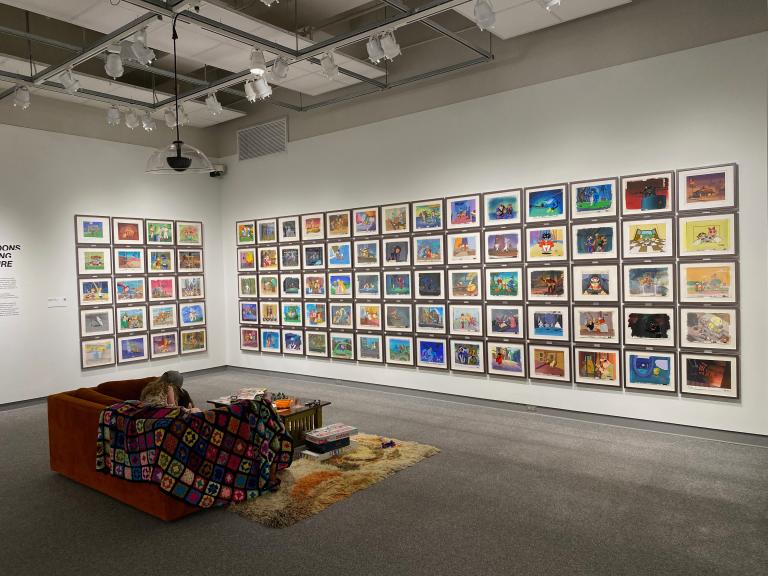The photograph captures a serene art gallery scene featuring two white walls adorned with a meticulously arranged grid of colorful animation cells from classic cartoons such as The Flintstones, The Jetsons, and Batman. The walls, one extending from the upper right to the center and converging with another that extends to the left side, display these 8x12 framed cells in neat, orderly rows against white mats inside gray frames. These vibrant pieces are a part of a larger installation in a museum-like space, characterized by a white ceiling sporting suspended lights on vertical rods. Below, a gray rug covers the floor, creating a gentle contrast to a vivid red sofa, which occupies the center of the room. The sofa is draped with a multicolored blanket on its right side, where a person with long hair and a gray ball cap sits, absorbed in the art display. In front of the sofa, a wooden coffee table with a glass top showcases various books and games. Adjacent to it, a brown and orange shag rug introduces a cozy texture beneath the person’s feet. The overall composition of the photograph highlights not only the vibrant art pieces but also the thoughtfully arranged furnishings that enhance the gallery’s inviting atmosphere.